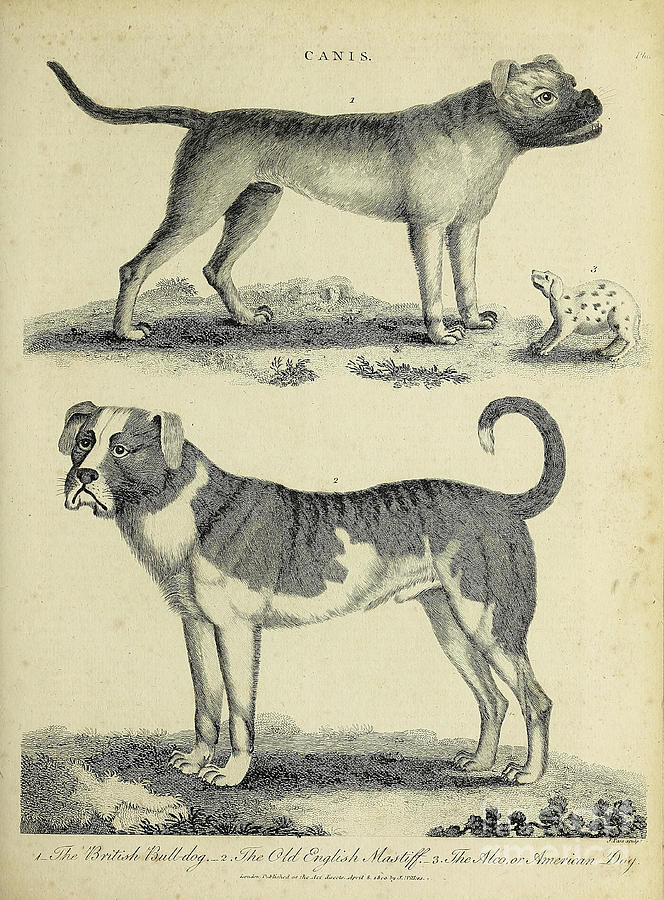This black and white sketch, possibly a photograph of an old, yellowed book page, depicts three dogs with the word "Canis" inscribed at the top in calligraphy. The primary dog in the illustration, facing right, has dark fur on its upper body that lightens towards its lower body. It has a sturdy, pit bull-like face, short floppy ears, and a long dark tail. Directly below this dog, a smaller dog cowers; this dog is light with dark spots, and its face and neck are predominantly white. Below them, another dog faces left, with its tail curled upwards. This third dog mirrors the fur pattern of the top dog, displaying darker fur above and lighter fur below. The scene is surrounded by visible age-related stain spots, adding to its antique charm. Although difficult to read, the text beneath the illustration appears to name different dog breeds in an ornate font.